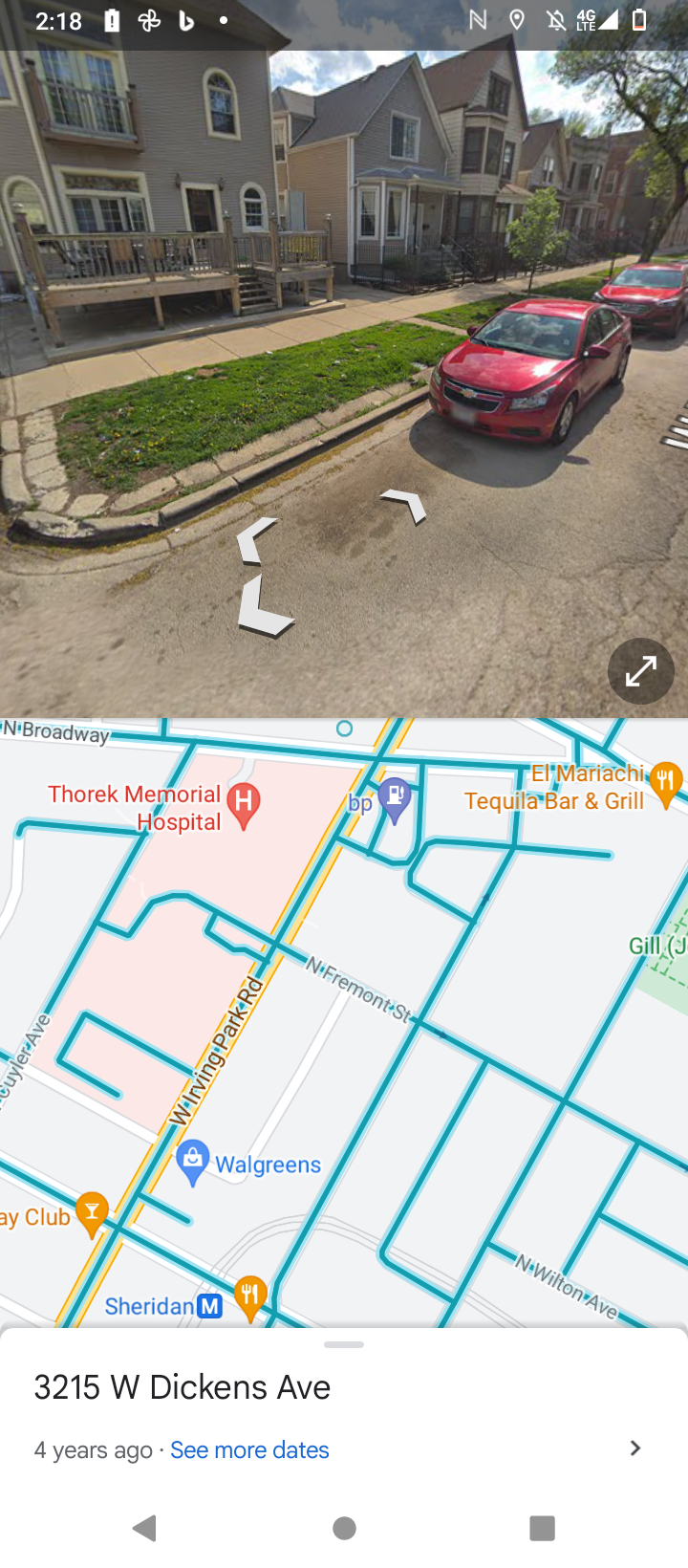In the top left corner of the image, there is an icon indicating the time as 2:18, along with battery status and notification symbols. Below this, a navigation map shows the address "3215 West Dickens Avenue" with a timestamp from four years ago. The map highlights several nearby streets, including North Fairmont Street, and landmarks like Toronto Hospital, Mariachi Tickle-by-and-grill, Walgreens, and Sheridan.

The main part of the image depicts a street view featuring multiple houses. On the left side of the road, there is a parked red car adjacent to a gray sidewalk. The street features directional arrows pointing to the left and upper right, indicating traffic flow. A green field is visible alongside the road. 

In the background, there is a gray building with multiple windows and a white railing. To the right, there is another house that is partly gray and brown. Additionally, there are several other houses along the street, including one that is notably blue. The scene captures a typical suburban setting with a mix of residential architecture and urban elements.